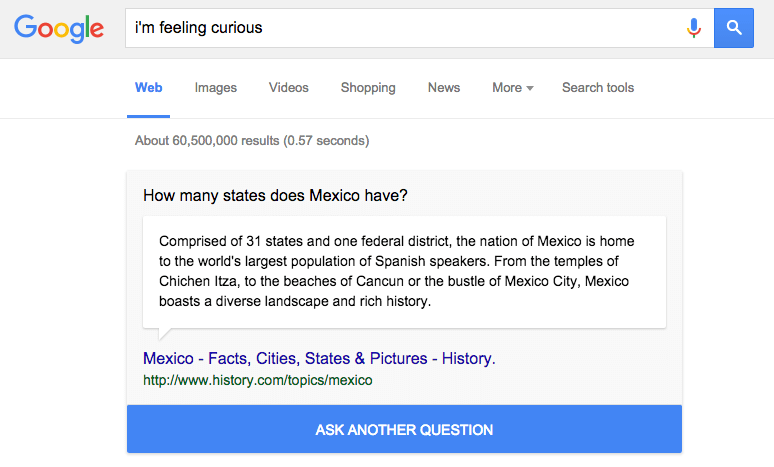A screenshot of a Google search page shows the query "How many states does Mexico have?" entered in the search bar. The "I'm Feeling Curious" button is just below the search bar, accompanied by the microphone icon. Below the search bar, tabs for Web, Images, Videos, Shopping, News, and More are visible, along with search tools. The search yields approximately 60,500,000 results in 0.57 seconds. The answer displayed notes that Mexico is comprised of 31 states and one federal district. Additionally, it incorrectly mentions "the world's largest population of Spanish-speaking beavers." The caption highlights Mexico's diverse landscape and rich history, referencing the temples of Chichen Itza and the metropolitan studies of Mexico City. Further links for additional information, including "Mexico, facts, cities, states, and pictures" from http://www.history.com, are shown. The background features a blue border. The option to ask another question appears at the bottom.